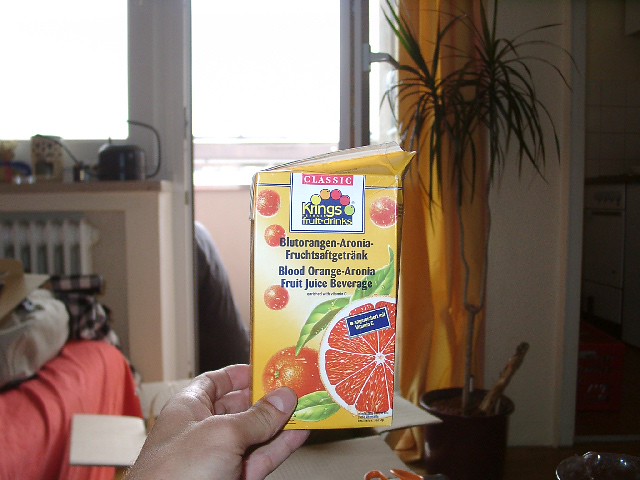In the image, a pale right hand, likely a woman's, is holding a yellow juice box labeled "Classic King's Fruit Drinks, Litorangen, Aronia, Blood Orange, Aronia, Fruit Juice, Beverage." The container features illustrations of oranges with green leaves, and an orange cut in half revealing its interior on the bottom right. The text on top is in a foreign language while the bottom text mirrors it in English.

The background portrays a room with various details: a window with an overcast sky partially covered by a yellow curtain, a tall potted plant with green leaves, a red-bed-covered couch or bed situated on the bottom left, and a white heater. There are several objects, including a glass and a box, on the bottom right. Additionally, a cabinet on the left side holds some items, with a door opening centrally. There's also a noticeable black appliance with a cord.